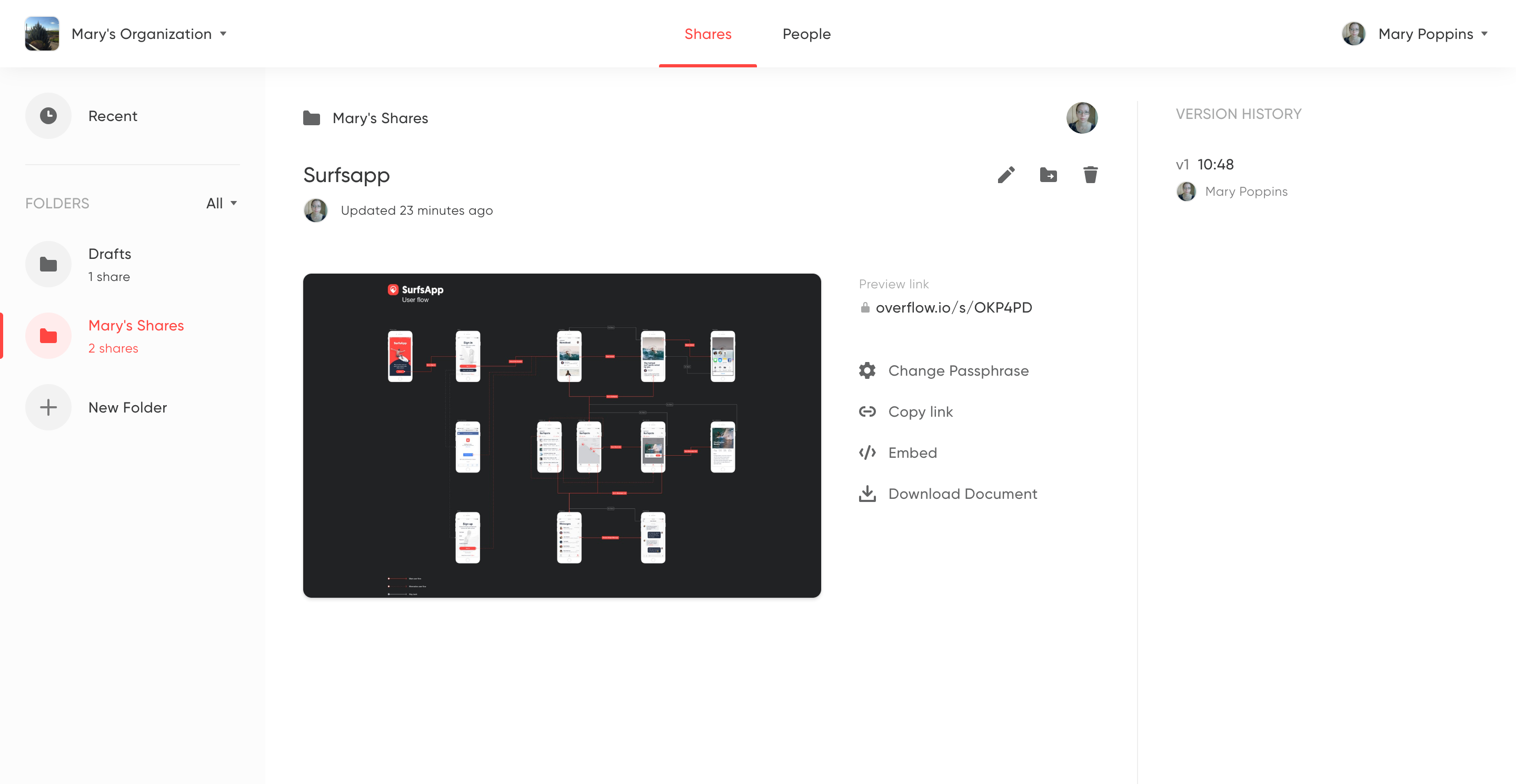The image portrays the interface of a web page, presumably for an organization named "Mary's Organization." At the top of the page, the header prominently displays "Mary's Organization" next to a small icon featuring a tree against a blue sky. To the right of this header, there are buttons for sharing and user interactions.

Beneath the header on the left-hand side, there is a navigation interface with various options. These options include "recent," followed by a section for folders. The folder section lists "drafts," "Mary's shares," and an option to create a "new folder."

On the main area of the page, directly to the right of these folder options, the label "Mary's shares" appears again, with the subheading "surfs app" beneath it. This section features an image depicting multiple phone screens interconnected by lines of various colors.

To the far right of the page, a vertical menu presents more options. These include "preview link" associated with overflow.io, "change passphrase," "copy link," "embed," and a button at the bottom labeled "download document."

Overall, the detailed layout indicates a comprehensive organizational tool, with various sections for managing and sharing documents and resources.